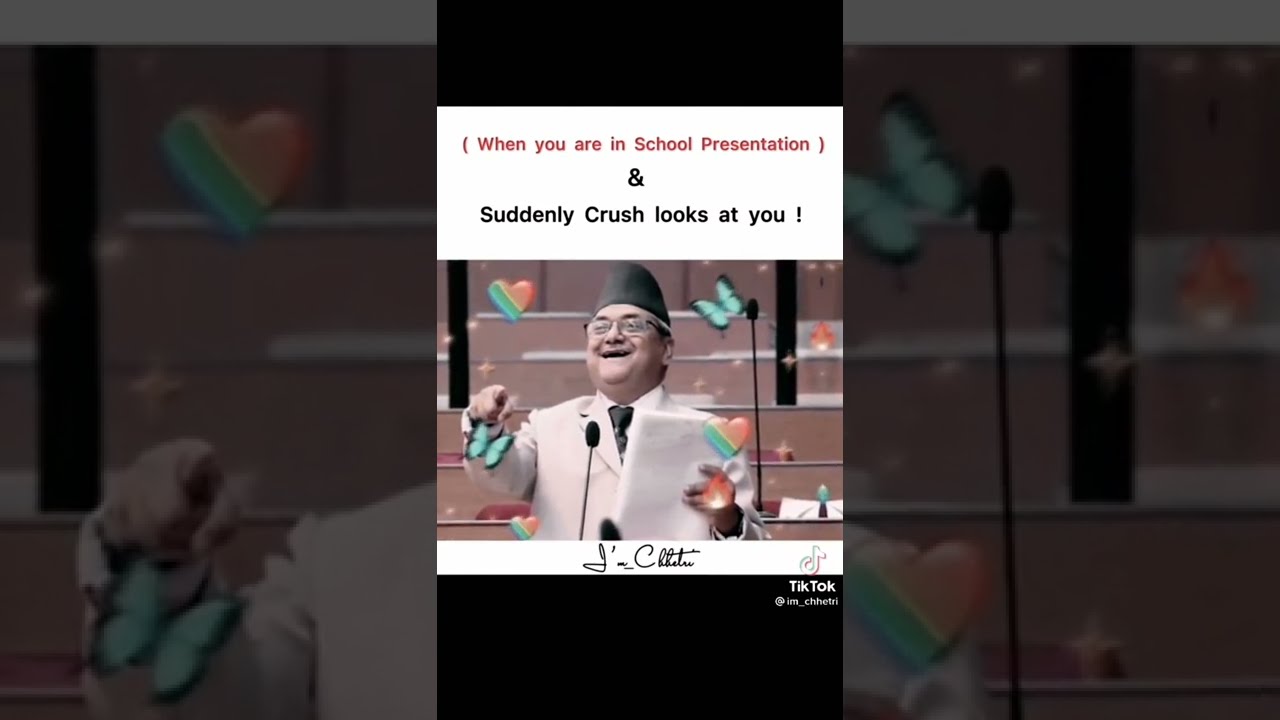The image is a horizontally rectangular screenshot of a TikTok video that features three panels. The central panel, slightly less than a third of the total width, displays a full-color photograph of an older man standing behind a microphone on a stand, situated indoors in front of some bleachers. He's wearing a light, pinkish-beige suit with a black tie, glasses, and a gray fez hat. He has his hands raised and is smiling goofily. The other two panels, on either side of the central image, are close-up, blown-up versions of the same photograph on a black, opaque background.

At the top of the central image, there’s a white bar with text in red and black: "When you're in school presentation and suddenly crush looks at you." The image has digitally imposed hearts and butterflies in various colors around the man, enhancing the whimsical and humorous nature of the meme. Below the main image is a signature, partially visible, reading "Jim C...". In the bottom right corner, there is a TikTok logo and a user handle, indicating it’s a TikTok meme.